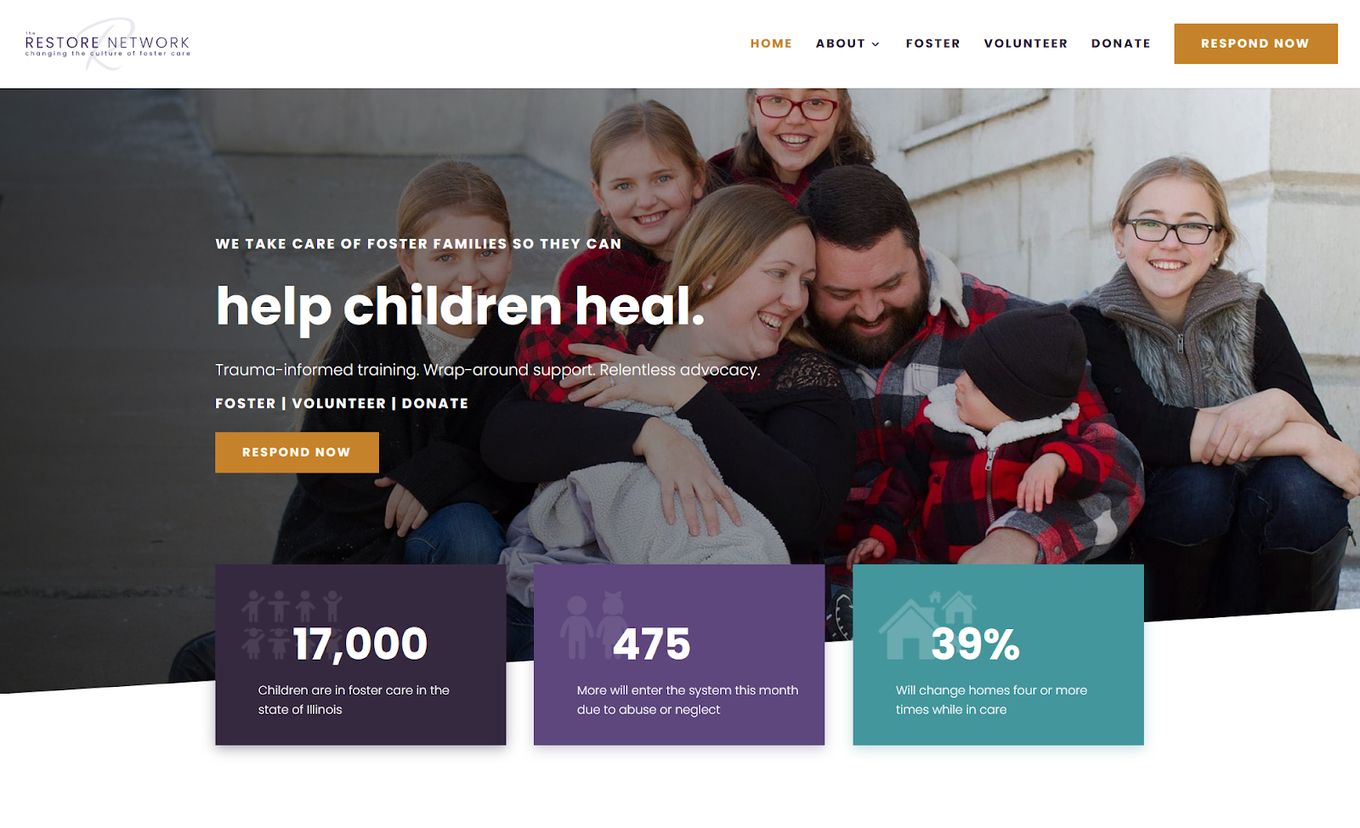Homepage of Restore Network: 

The top section features a clean white background with black text stating "Restore Network: Changing the culture of foster care." 

Centered at the top is an orange menu with "Home," followed by black text options for "About" (with a dropdown menu), "Foster," "Volunteer," and "Donate." An orange rectangle with white text reading "Respond Now" is prominently placed at the upper right corner. 

Below, a large, rectangular image depicts a Caucasian family consisting of two parents and approximately six children. Of the seven individuals, five are female, two are male, and one child is an infant.

Overlaying the photo on the left side in white text is the message: "We take care of foster families so they can help children heal." Below this are the key service areas: “Trauma Informed Training, Wraparound Support, Relentless Advocacy.” Further down, the options to "Foster," "Volunteer," and "Donate" are listed, followed by another orange rectangle with the call to action "Respond Now."

The footer contains three distinct colored rectangles:
1. The first rectangle is a gray-purple-gray with white text that reads, "17,000 children are in foster care in the state of Illinois."
2. The middle rectangle is purple with white text stating, "475 more will enter the system this month due to abuse or neglect."
3. The final rectangle is light blue with white text declaring, "39% will change homes four or more times while in care."